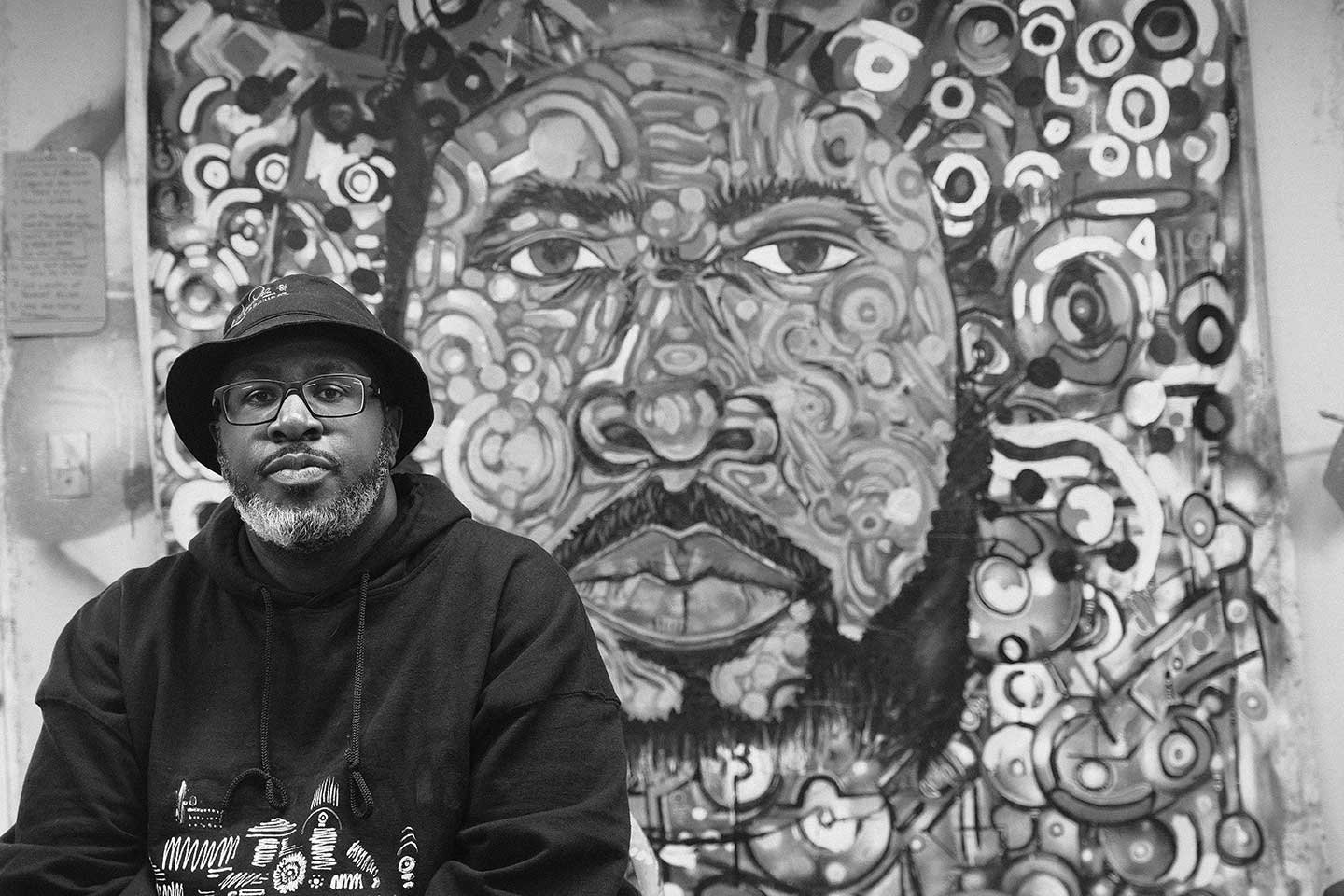In this high-quality black-and-white photograph, a dark-skinned man with a bucket hat bearing white lettering and transparent glasses sits front-facing towards the camera. He has a graying beard, with a solid black mustache and the rest of his beard completely gray. Dressed in a black hoodie adorned with various white squiggly symbols and strings hanging down the front, he sits against an intricate mural. The mural behind him depicts a similarly dark-skinned man whose face is crafted from numerous white and black circles and swirls, making it appear remarkably realistic. While the mural subject does not wear glasses or a bucket hat and has a solid gray beard and mustache, they share a striking resemblance. To the top left of the mural, a plaque is visible, likely detailing its significance. The image has a professional feel, capturing both the individual and the mural in a detailed and cohesive composition.